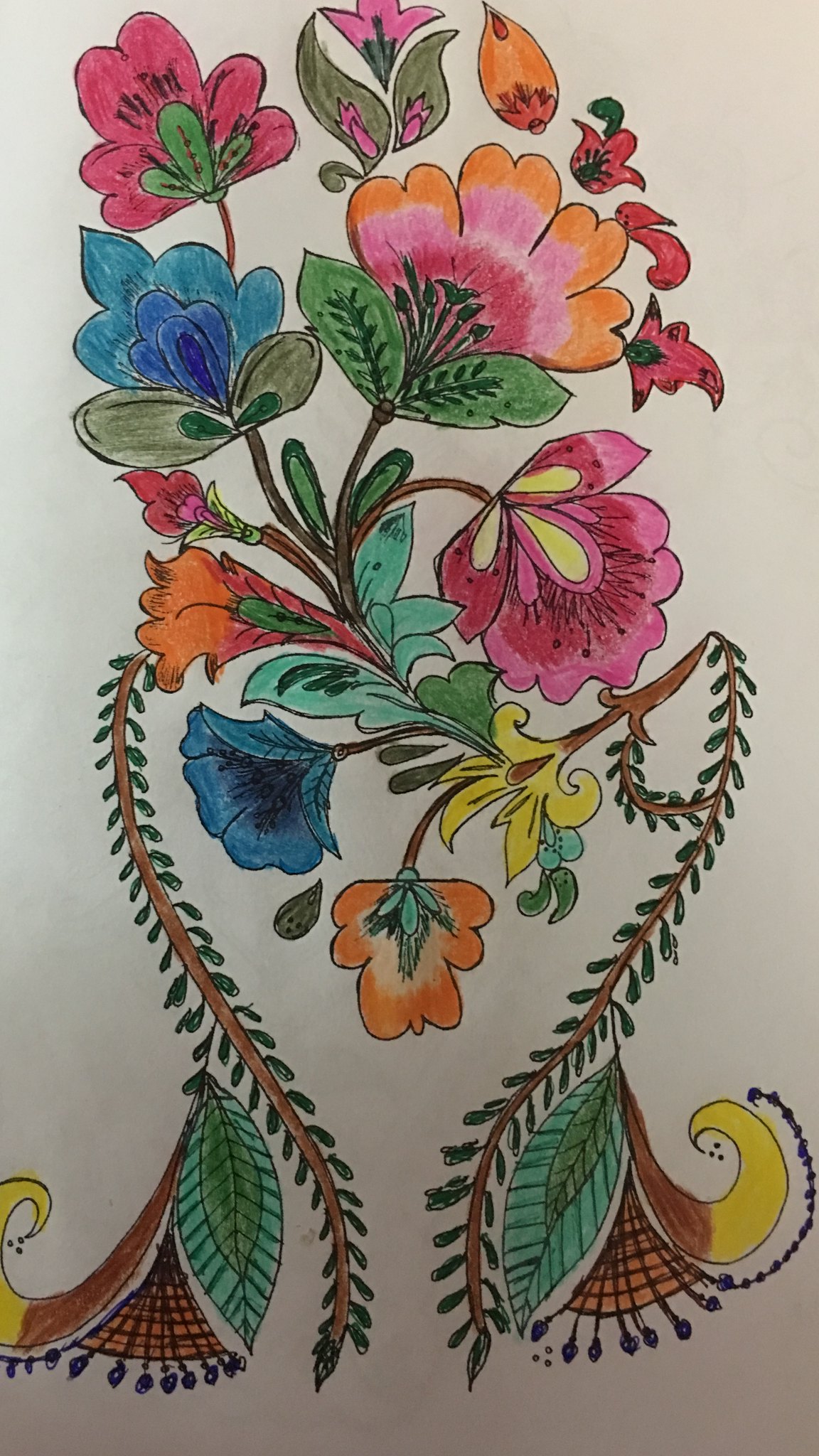This image showcases a detailed and vibrant artwork of flowers and plants on a stark white background. The composition features an array of colorful flower petals and ferns, which collectively create a heart-shaped formation with the flowers situated in the lower half of the image. The top section prominently displays flowers with varying hues: a red flower with a green center on the top left, a blue flower with light blue petals transitioning to darker blue and an olive and dark green core just below it, and a striking multicolored flower on the right with orange tips, transitioning through pink and red, and a dark green center. Smaller red flowers are scattered around the central arrangement. Additional details include two fern leaves arching gracefully from above, contributing to the heart shape, and a large leaf surrounded by brown and yellow swirls. The artwork is rendered in a style reminiscent of colored pencil drawings, exuding a vibrant, yet simple charm.